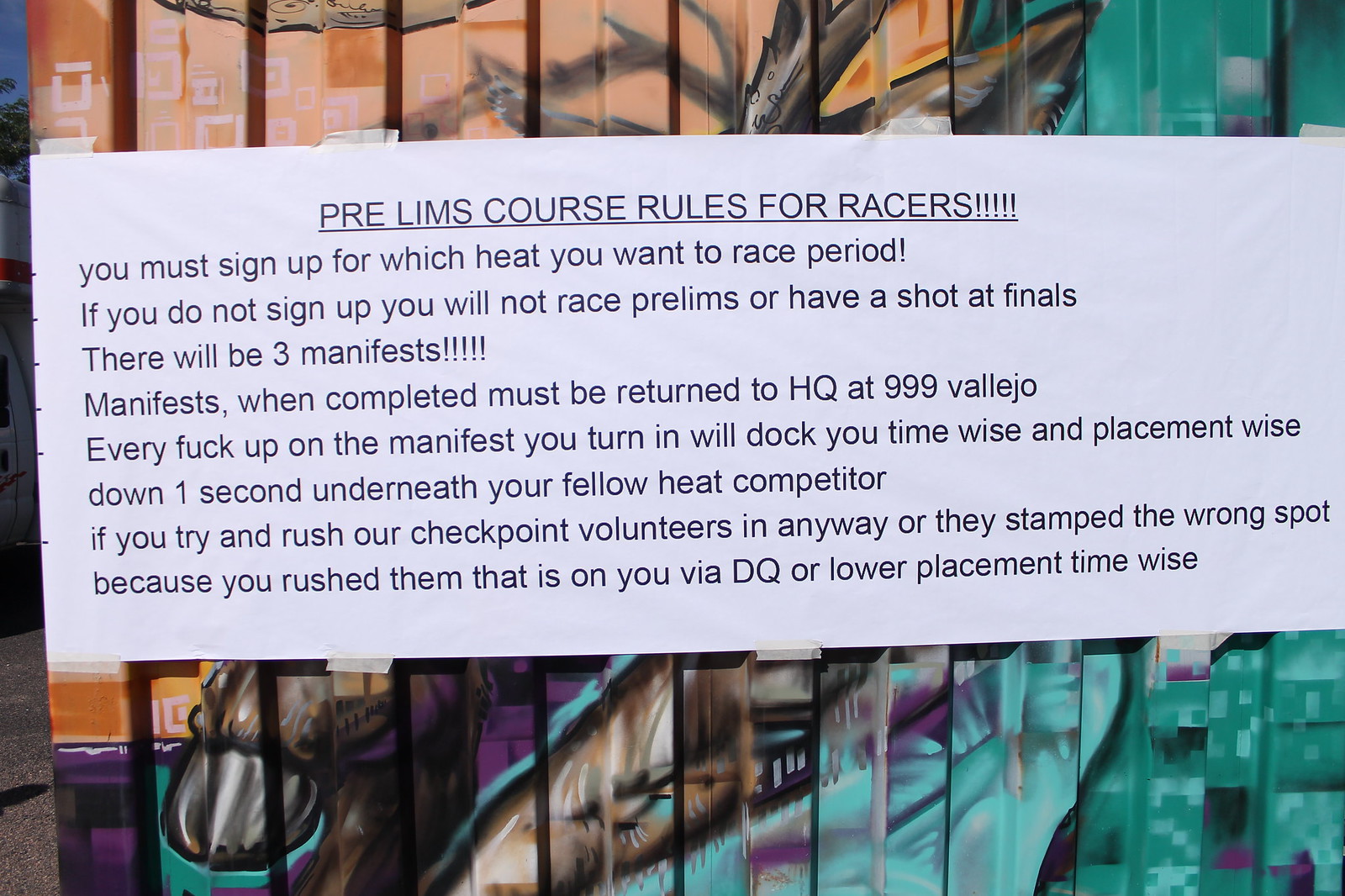The photo captures an outdoor scene featuring a vividly graffiti-painted wall with vertical sections in varying colors: orange on the top left, brown in the center, and turquoise on the top right and bottom. Affixed to this wall is a large, horizontally rectangular white paper with black text. The upward background reveals a glimpse of blue skies, trees, and a nearby building with asphalt visible at the ground level. The paper, taped prominently on the wall, displays the "Prelims Course Rules for Racers" in capital letters, underlined at the top. The detailed rules stipulate that racers must sign up for their heat; failure to do so will result in disqualification from the prelims and finals. It also mentions that three manifests must be completed and returned to HQ at 999 Vallejo. Any errors on the manifest will result in a one-second time penalty per mistake, compared to fellow competitors. Furthermore, the notice warns that rushing checkpoint volunteers, which could lead to incorrect stamping, will result in disqualification or lower placement times.